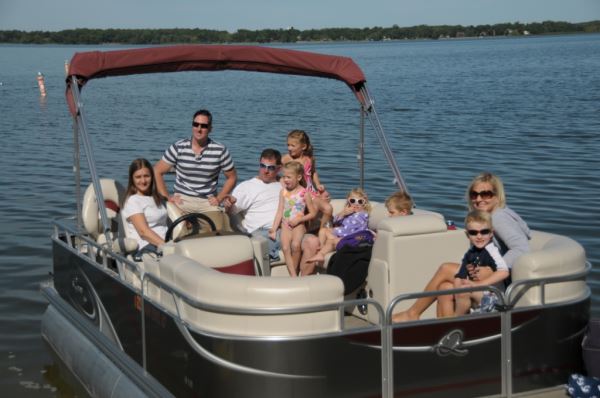The image depicts a large family on a anchored boat enjoying a leisurely day on a bluish-gray body of water, under a sky that appears cloudy. The boat is a horizontally-aligned rectangle with dark brown sides and a gray bottom, featuring off-white or beige-colored seats. 

The background shows a strip of trees and houses across the horizon, with the majority of the setting dominated by gently rippling water.

Within the group, three adults can be seen, all wearing sunglasses. One man, dressed in a blue and white striped collared shirt and tan khaki pants, is standing at the edge of the boat. Another man, outfitted in a white t-shirt and blue denim pants, is seated towards the back. A woman in a gray sweatshirt is holding a little boy in the back right corner, and there is a teenage girl at the steering wheel, although it looks like the boat is stationary.

There are five children in the photo: one girl sitting on the lap of the man in the striped shirt, another behind him, and a third to his side, all in swimsuits, along with a child with the woman in the sweatshirt. The overall scene captures a relaxed family outing, with everyone contentedly enjoying their time on the water.